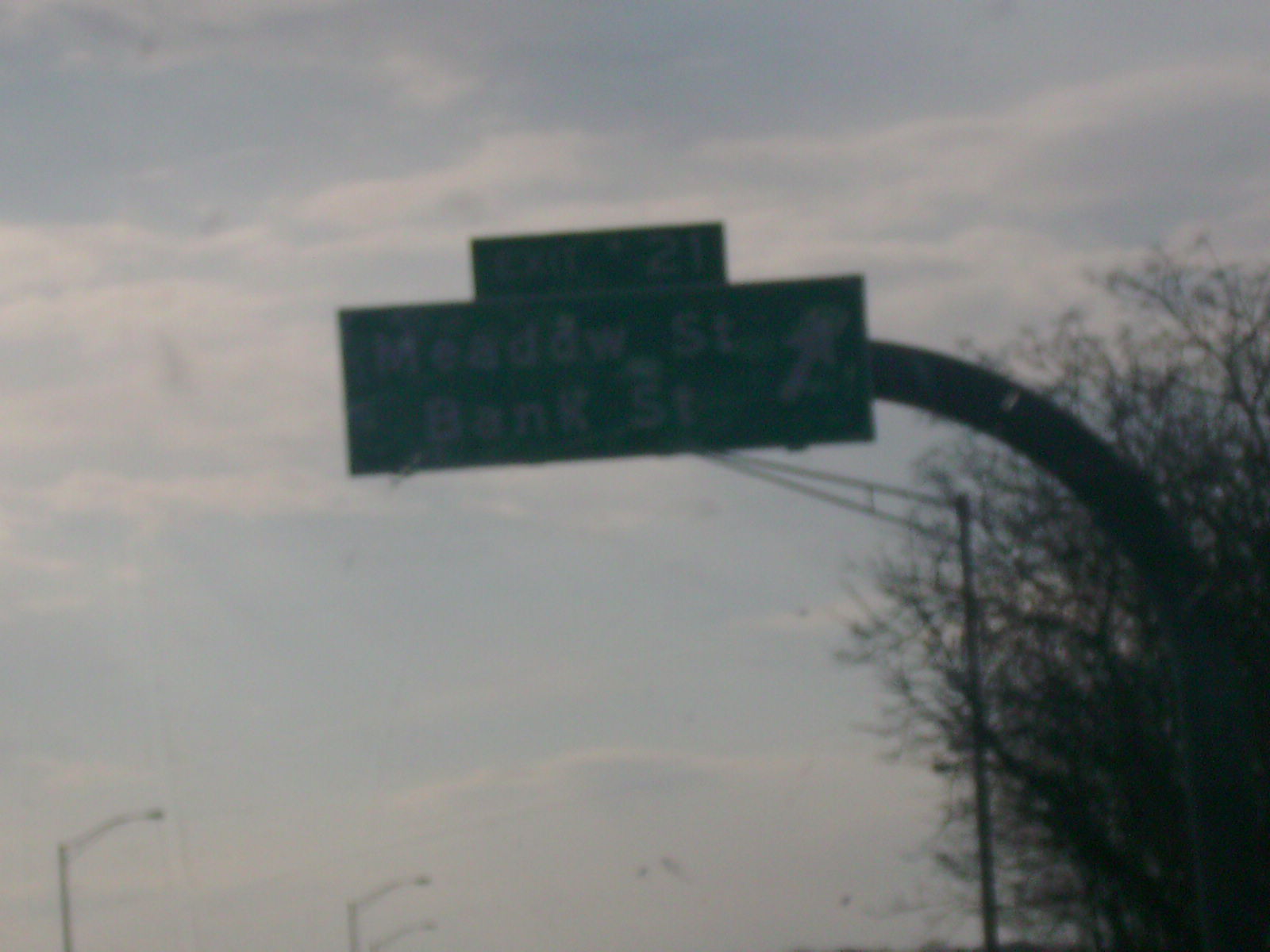This image features a highway sign prominently mounted on a large metal pole, extending over the road. The sign indicates "Exit 21 Meadow Street and Bank Street" with an arrow directing to the upper right. The quality of the photo is somewhat compromised, appearing fuzzy with gray and dull lighting, suggesting a possible overcast day. Despite the mediocre quality, a blue sky with some scattered clouds is visible in the background. To the right side of the image, there is a large tree devoid of leaves, showing only barren branches, which hints that the photo was likely taken during the fall season.